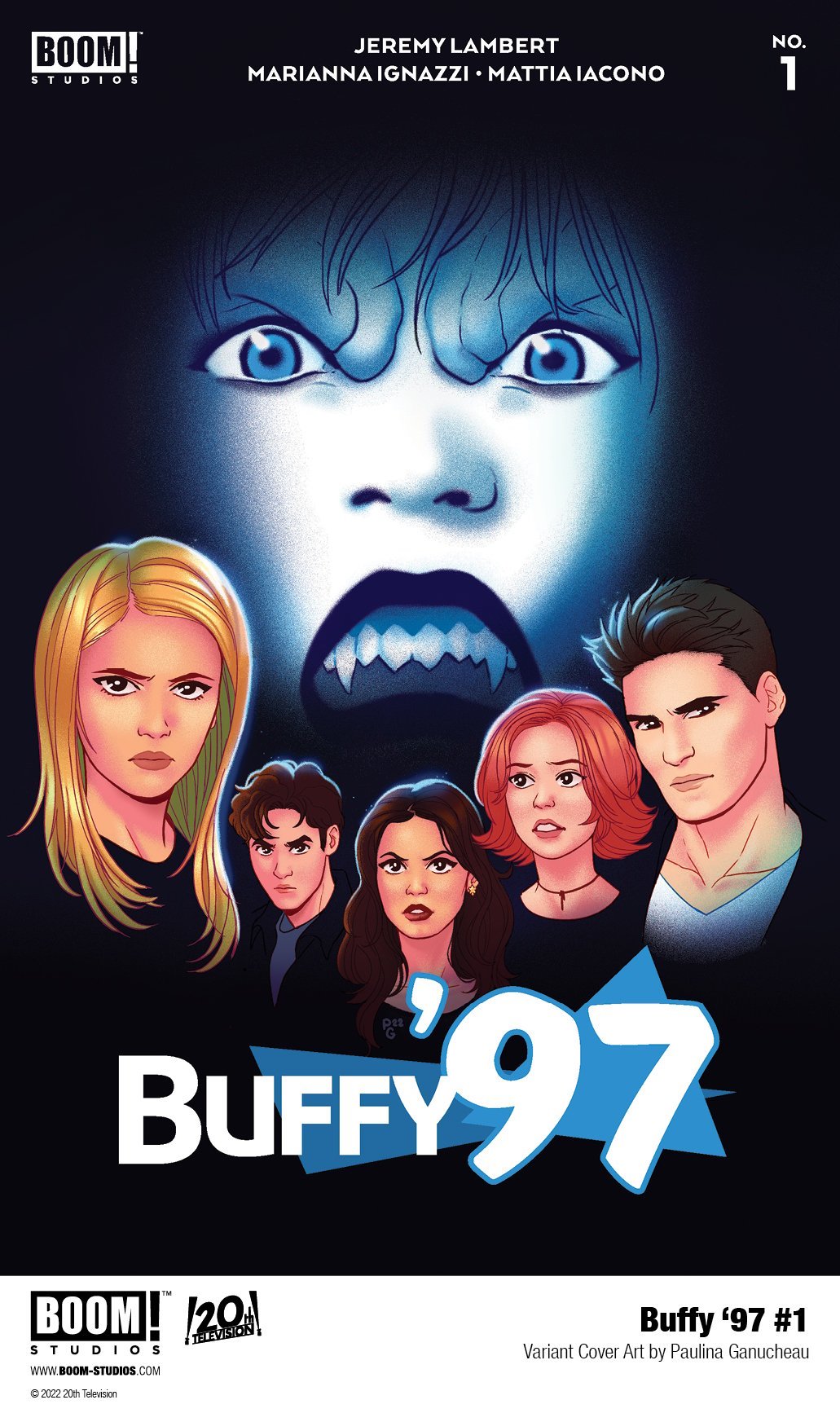This poster for "Buffy 97," either a show or a movie, features a detailed and striking computer-generated image. Dominating the background is a large, eerie vampire face with fangs, rendered in blue-white hues, her mouth open in a frightening expression. Below this menacing figure, five characters are positioned, all gazing seriously in the direction of the viewer. The characters include a blonde-haired woman, a man with brown hair, a brunette woman looking intently, an orange-haired woman glancing to the side, and a man with short black hair. At the top of the poster, the names Jeremy Lambert, Mariana Ignazi, and Mattia Iacono are displayed prominently. "Boom Studios" is noted in the top left corner, and "Number One" is in the top right. At the bottom of the poster, the title "Buffy 97" is featured, with additional information provided beneath. The background of the characters is black, which enhances the stark contrast with the blue vampire and the overall dramatic effect of the poster.